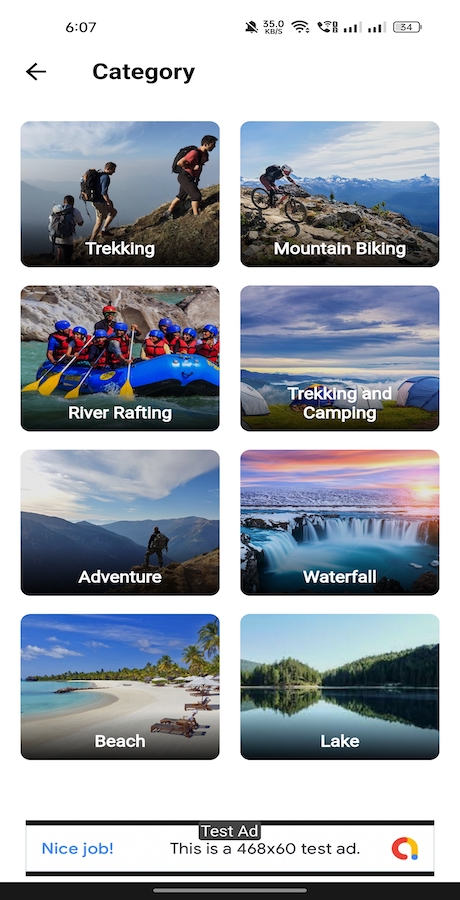This is a detailed caption for the provided image:

---

In the screenshot, sourced likely from a travel app on an Android phone, the clean white background emphasizes the app's interface. The top of the screen features standard status icons from the Android operating system: the time showing 6:07 on the left, followed by the Wi-Fi signal icon, mobile data icon, and battery percentage icon.

Just below this status bar, the app's interface begins. The word "Category" appears in black text towards the top left, accompanied by a left-facing arrow at the very top left corner indicating a back navigation option.

The main content of the screenshot is a grid of eight boxes, each showcasing a different adventure activity with a corresponding image. These boxes include:

1. "Trekking": An image of people trekking in nature.
2. "River Rafting": A picture of individuals rafting in a small blue raft.
3. "Adventure": A dramatic image of a person standing triumphantly on a mountaintop.
4. "Beach": An image showcasing a serene beach scene.
5. "Mountain Biking": Depiction of a person biking through rugged terrain.
6. "Trekking and Camping": A scenic image of an open ground with several tents set up.
7. "Waterfall": A beautiful image of a cascading waterfall.
8. "Lake": A tranquil image of a picturesque lake.

At the bottom of the screen, there's a small banner displaying a test ad. The banner text reads, "Nice job! This is a 468x60 test ad."

---

This caption provides an organized and detailed description of the screenshot, highlighting each element clearly.